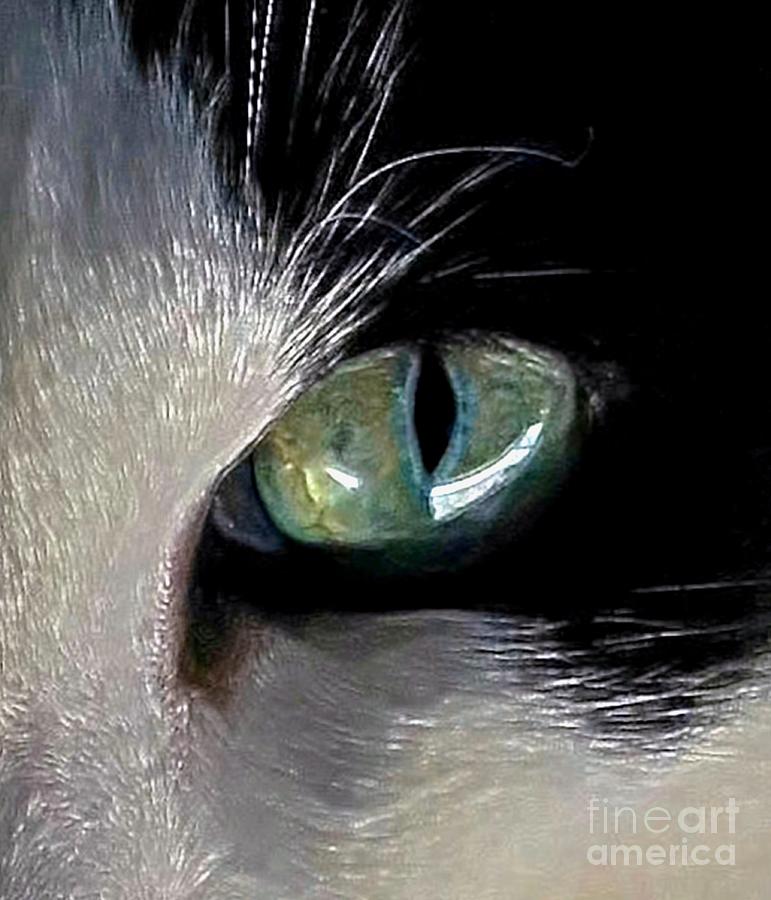The image depicts an extreme close-up of an animal’s right eye, likely a cat or a tiger, given the detailed descriptions of the fur and eye features. The eye itself is green with a vertically oriented black iris, surrounded by a black outline along the eyelid. There's a prominent presence of white fur, particularly around and beneath the eye, extending to cover part of the nose's top but not revealing the nostrils. The fur includes some longer hairs sticking out sporadically. The background appears dark, almost black, giving a stark contrast to the animal's eye and fur. The entire composition is tightly framed, falling between the dimensions of a square and a rectangle, making the eye the focal point of the image.